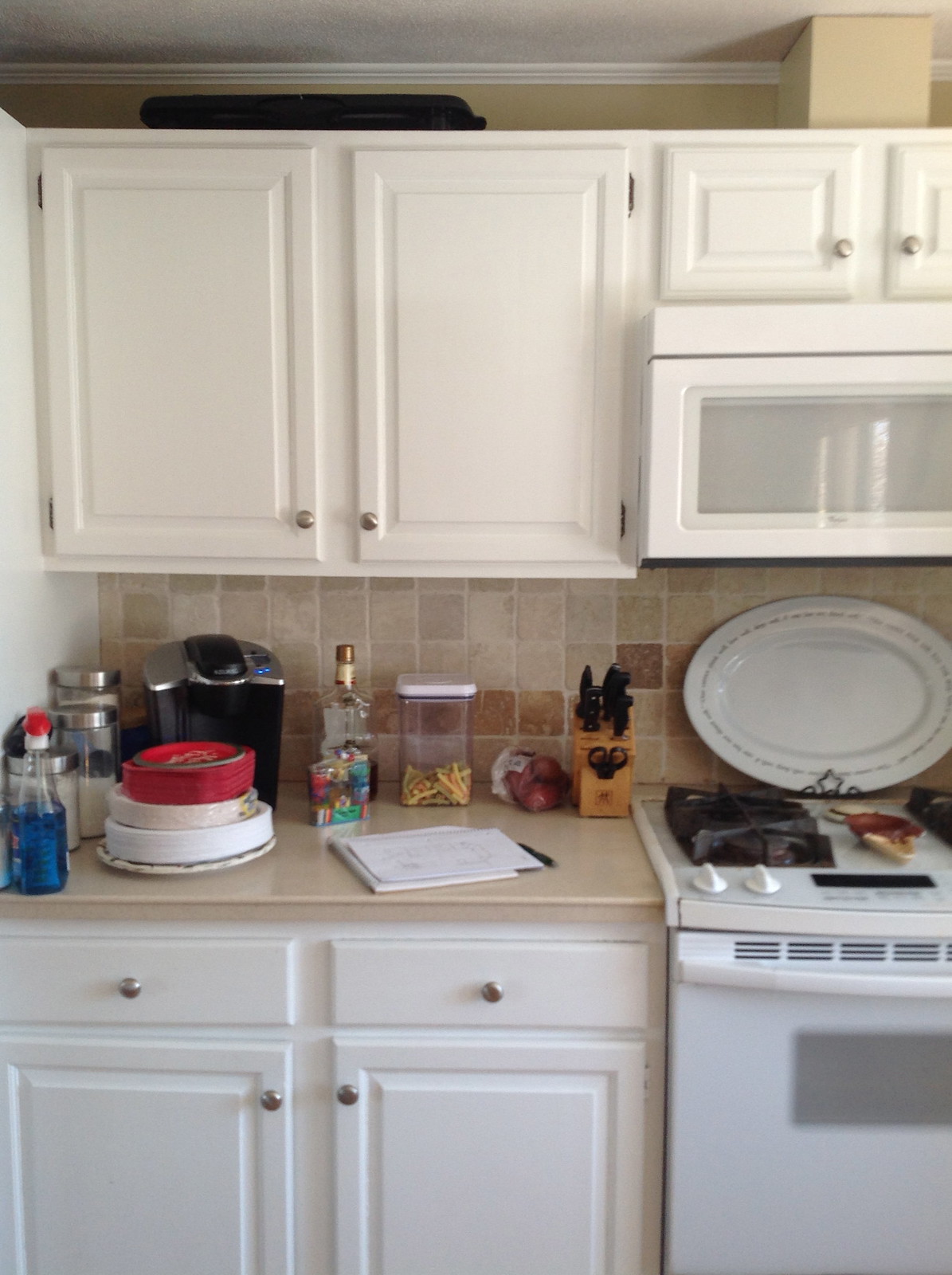The image depicts a detailed view of a kitchen interior. On the right side at the bottom, half of a white stove is visible with two buttons on the front left side and two black burners above these buttons. In the center of the stove, there's a brown item with a gradient to a lighter brown towards the front. A small corner of an additional burner is peeking in. Below the stove handle is a small opening into the dark interior of the stove. 

To the left of the stove, there are two small drawers with another off the left edge of the image. Below these drawers, there are two cabinet doors that open outward, with the left door opening to the left and the right door to the right. The knobs are located in their corresponding corners, with an additional knob in the center of the small drawers above.

Above this cabinetry is a brown countertop cluttered with various items: jars, a pile of plates on the left side, a black coffee pot with a silver top, a bottle, some white papers at the bottom of the countertop, a plastic container with a white lid, a small bag of fruit, and a knife block. The backsplash behind this area is made of linoleum with squares in shades of brown, orange, and dark brown.

Above the stove, leaning against the wall, is an oval-shaped white plate. At the top of the image, there's a white cabinet with two large doors; the left door's handle is at the bottom right corner and the right door's handle is at the bottom left corner. Adjacent to this is another set of double doors at the top, with a microwave installed just below them. The handles of these top doors are positioned in the bottom left and right corners, respectively.